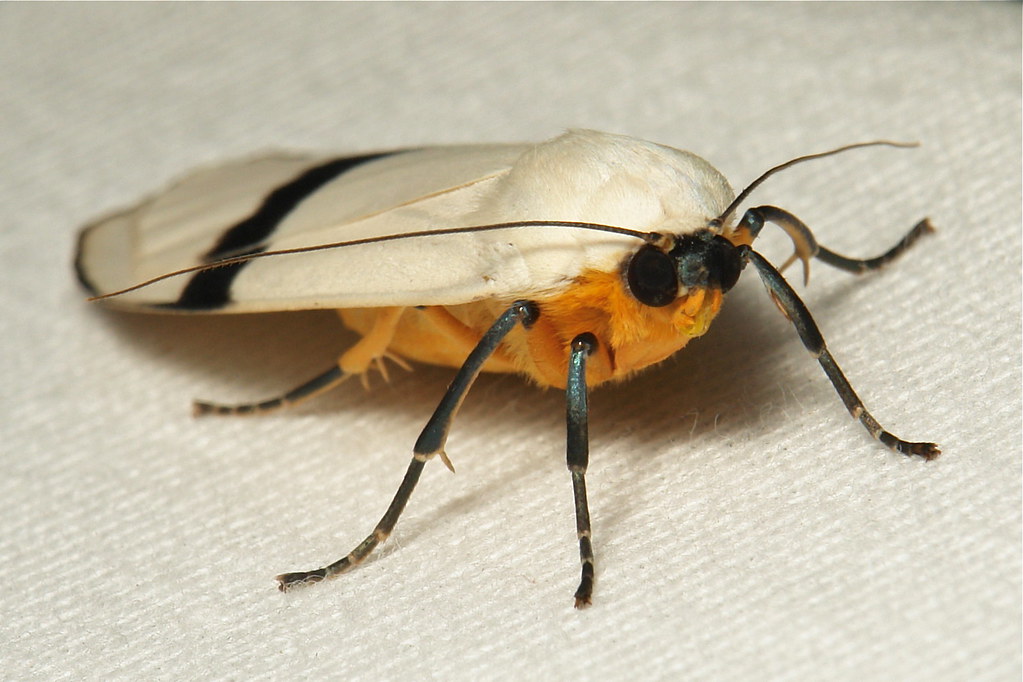The image is a highly detailed close-up photograph of a large moth resting on a textured white surface, likely a paper towel. The moth itself, approximately two inches in length, is positioned diagonally with its head facing the bottom right corner and its wings extending towards the top left. The moth’s body is a fuzzy goldish-yellow or orangish color, and it has five visible black legs, with the rear leg partially orange. Its wings are closed, forming an oval shape, and are primarily white with a distinct black stripe near the bottom. The moth has two small black eyes and long antennae extending above them, and the overall texture and fuzziness of the moth are clearly visible in the image.